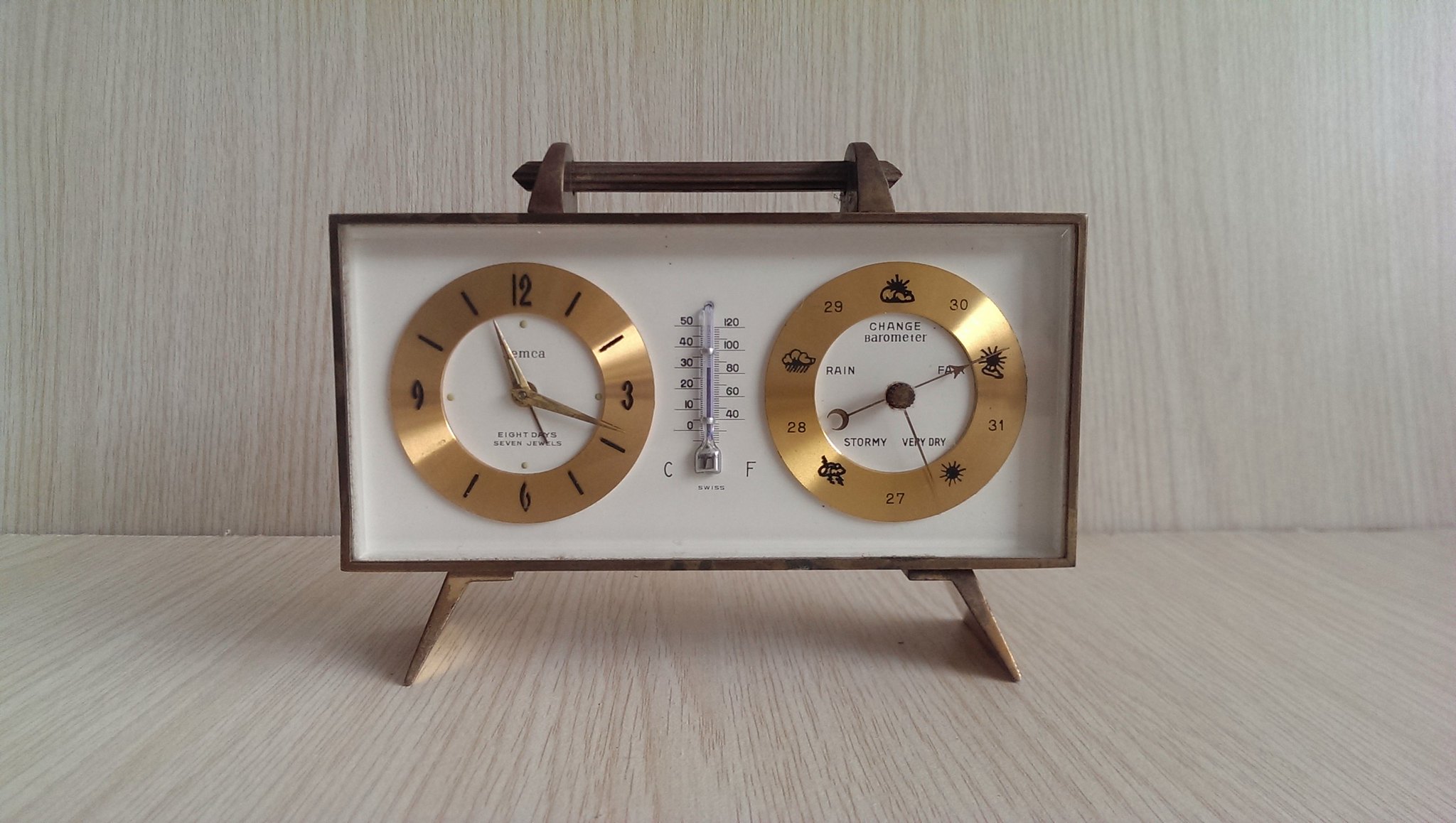The color landscape photograph showcases a vintage device from the late 40s or early 50s, featuring a clock, barometer, and thermometer, all encased in a rectangular wooden frame. The photograph is taken indoors, with the device set against a light-colored wooden surface, creating a harmonious background and foreground. The wooden case has a handle at the top and two diagonally extending legs at the bottom for support.

On the left side of the case is a clock with a gold ring face, displaying the numbers 12, 3, 6, and 9, while the remaining time markings are indicated by hash marks. The gold clock hands show the time as around 11:17, with the second hand pointing to the 5. Centrally placed within the configuration is a mercury glass-filled thermometer, marked with both Celsius and Fahrenheit scales, showing a temperature of about 75 degrees.

To the right of the clock is the barometer, set in an identical gold ring. The barometer face is labeled "CHANGED BAROMETER" and displays a range of measurements from 27 to 31, with additional indications of weather conditions like "Very Dry," "Stormy," and "Rainy." The barometer has two arrows: one black arrow pointing towards an image resembling planting, and another arrow pointing to the "Very Dry" marker.

The entire arrangement is meticulously crafted, with the warm tones of the wooden casing and the gold details of the instruments complementing each other beautifully, evoking a sense of nostalgia and classic design.